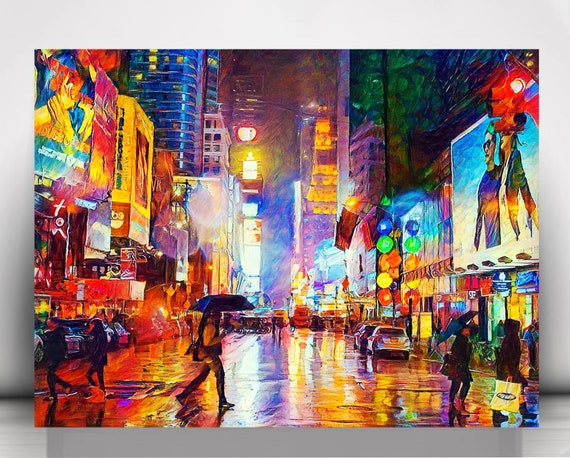The image is a striking, vibrant painting of a modern city street at night, bathed in the glow of neon lights and illuminated advertisements. The urban scene, reminiscent of districts in Japan or a futuristic landscape out of Blade Runner, captures the essence of a rainy night with reflections of various bright colors dancing on the wet tarmac. Starting from the bottom left, the street transitions through a spectrum of reddish hues, blues, and yellows. The road is adorned with parked cars; two on the right-hand side and a queue of vehicles on the left. People with umbrellas and shopping bags navigate the bustling street, adding to the lively atmosphere. Above the shop fronts, an array of colorful billboards and advertisements lights up the scene, extending the illumination further down to the buildings in the background. The image is a mesmerizing collage of light and color, depicting a cheery yet wet urban nightscape full of life.